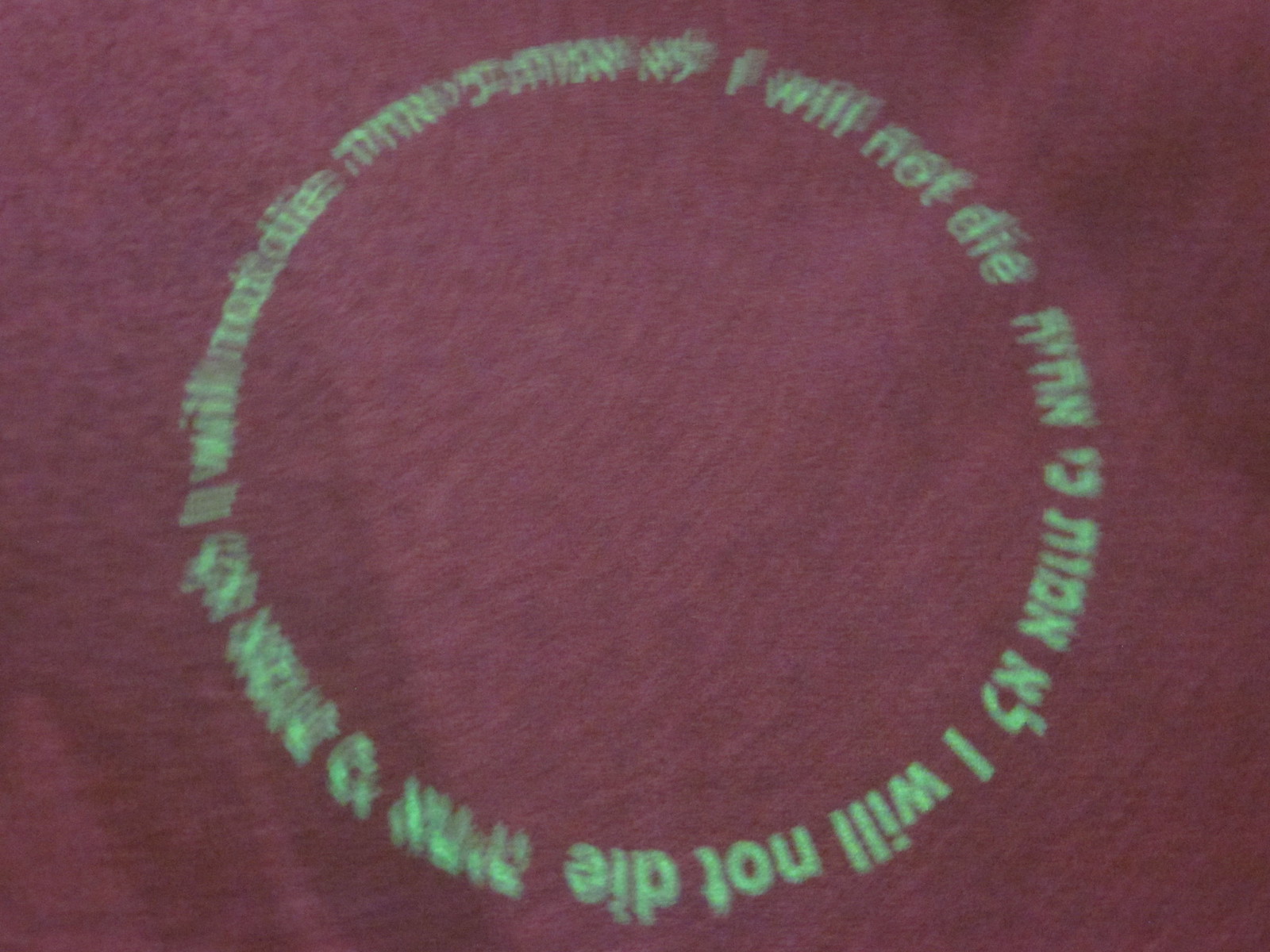The image is a close-up of a burgundy t-shirt featuring a circular graphic with greenish-yellow text that reads "I will not die." This phrase is repeated in a circular pattern interspersed with words or symbols in Hebrew, likely echoing the same sentiment. The graphic design is prominent on the front of the t-shirt, and the detailed text contrasts sharply with the t-shirt's rich maroon background. The image is somewhat blurry, which adds to the challenges of distinguishing the exact details of the Hebrew symbols.